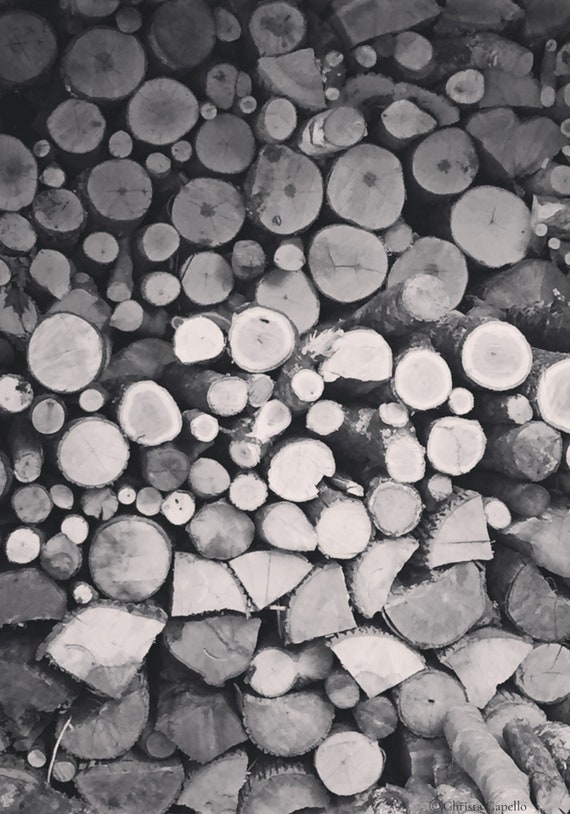This monochrome black and white photograph, wider than it is tall, captures the neatly stacked end of a large pile of firewood, ideal for a wood-burning stove or fireplace. The firewood is arranged in approximately 16 compact layers from bottom to top. The lower section features larger, round trunks and branches cut to manageable sizes, forming a solid base. Above this, there are half-circular pieces created from split logs alongside quartered triangular pieces resembling pie slices. Ascending higher, the stack is interspersed with various sizes of smaller round branches and trunks, creating a textured and organized pattern. The entire composition is viewed straight on, revealing the meticulous stacking that includes some wood pieces as round as the palm of a hand. At the bottom right corner, a small, darker gray watermark reads "copyright Krista Capello" in fine print.